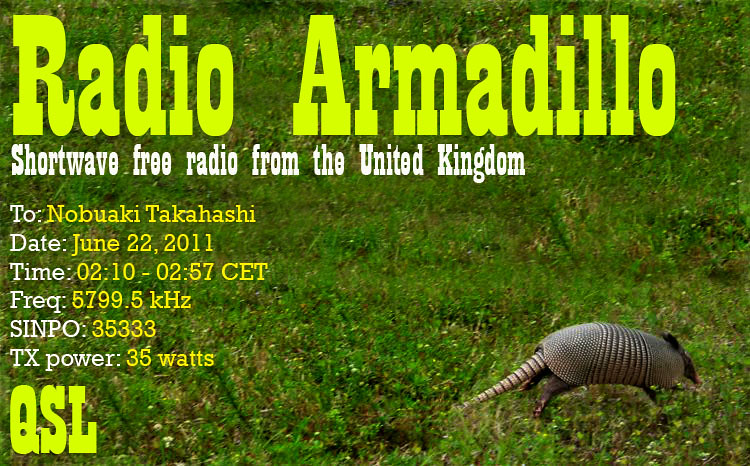This photograph features an armadillo, prominently positioned against a backdrop of open green space, suggesting a natural, meadow-like environment. The armadillo, a small to medium-sized animal with a long tail and an appearance akin to wearing chain mail, looks as if it is leaping into the greenery. This image serves as an advertisement for "Radio Armadillo," a shortwave free radio station from the United Kingdom. Text details in the image include broadcasting specifics: "June 22, 2011" addressed to "Nubiaki Takahashi," and the times listed are from "210 to 257 CET." Additionally, it highlights the frequency "5799.5 kilohertz," the signal's SINPO rating, and a transmission power of "35 watts." The cohesive theme ties the armadillo's imagery to the radio's name, playing on visual and linguistic elements.